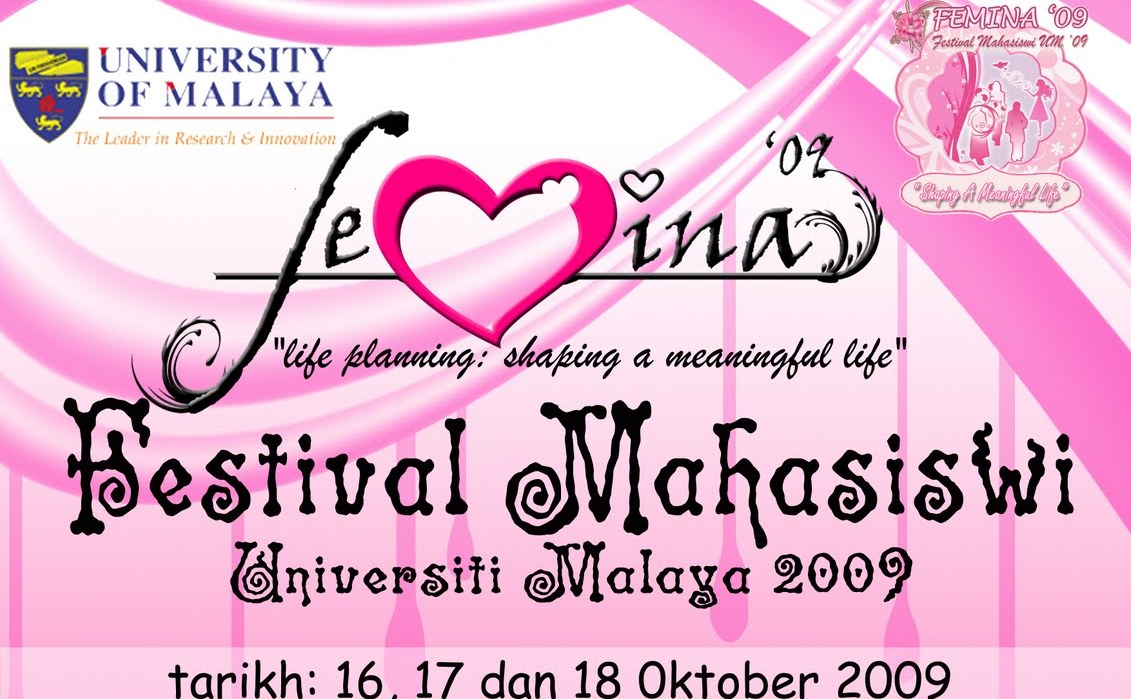The image features a vibrant pink, white, and purple background. In the top left corner, it prominently displays the logo of University of Malaya alongside the text "The Leader in Research and Innovation." The emblem, which consists of a blue shield adorned with three yellow lions and additional yellow and red elements, is centrally placed. In the top right corner, the word "Femina" appears in a striking combination of black letters and a pink heart symbol, indicating the festival's name. Below this, detailed information follows in smaller fonts: "Life Planning, Shaping a Meaningful Life, Festival Mahasiswi University of Malaya, 2009." Additionally, the dates "Tariq 16, 17, and 18 October 2009" are noted at the bottom. The overall design suggests it's a promotional sign for a life-planning festival organized by the university.